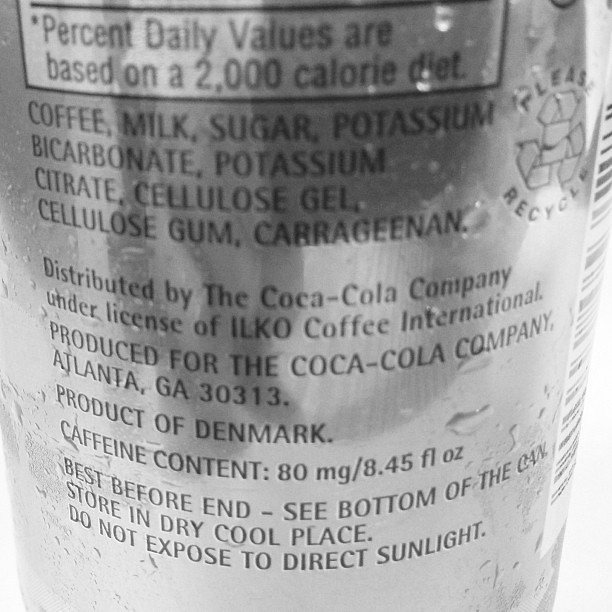This close-up black-and-white photograph captures a soda can produced by the Coca-Cola company in Denmark. The silver, reflective surface of the can glistens with dots of condensation. A small light gray rectangle at the top reads, "Percent daily values are based on a 2000 calorie diet." Below this, the ingredients are listed in black text, including coffee, milk, sugar, potassium bicarbonate, potassium citrate, cellulose gel, cellulose gum, and carrageenan. The text further details that the product is distributed by the Coca-Cola company under a license from Isklo Coffee International and produced for the Coca-Cola company in Atlanta, Georgia, ZIP code 30313. The caffeine content is specified as 80 milligrams per 8.4 fluid ounces. Additional instructions advise storing the can in a dry, cool place and avoiding direct sunlight. Towards the right side of the can, a white rectangle with black stripes serves as the UPC code, next to which a recycling symbol accompanied by the words "please recycle" is visible. The bottom of the can indicates its best-before date.